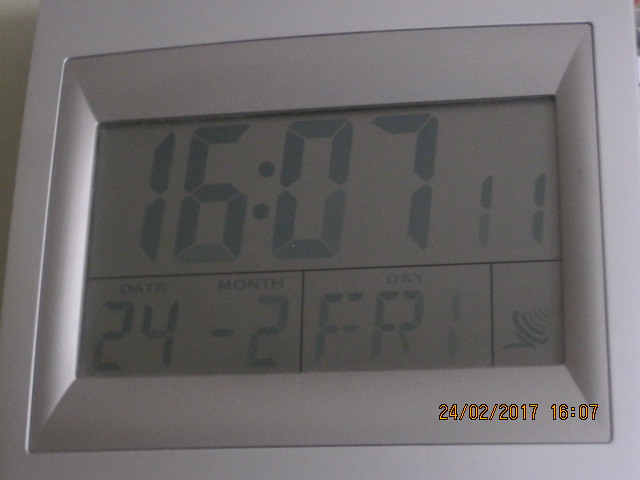This close-up photograph captures a sleek, metallic aluminum digital clock. The clock's rectangular body features a smooth, reflective metallic surface with an inset that houses a monochromatic black and white screen. Dominating the upper 60% of the screen, the time is clearly displayed as 16:07:11. Below the time, the screen is divided into three distinct boxes that present additional information: the date "24-02" (day-month format), the day "Friday," and an indicator symbol that suggests Wi-Fi connectivity.

In the lower right corner of the clock, there's a small, gold-colored watermark detailing the photo's timestamp, reading "24-02-2017" and "16:07," presumably added by the camera used to capture this image. The overall design of the clock is modern and functional, emphasizing clear readability and connectivity features.